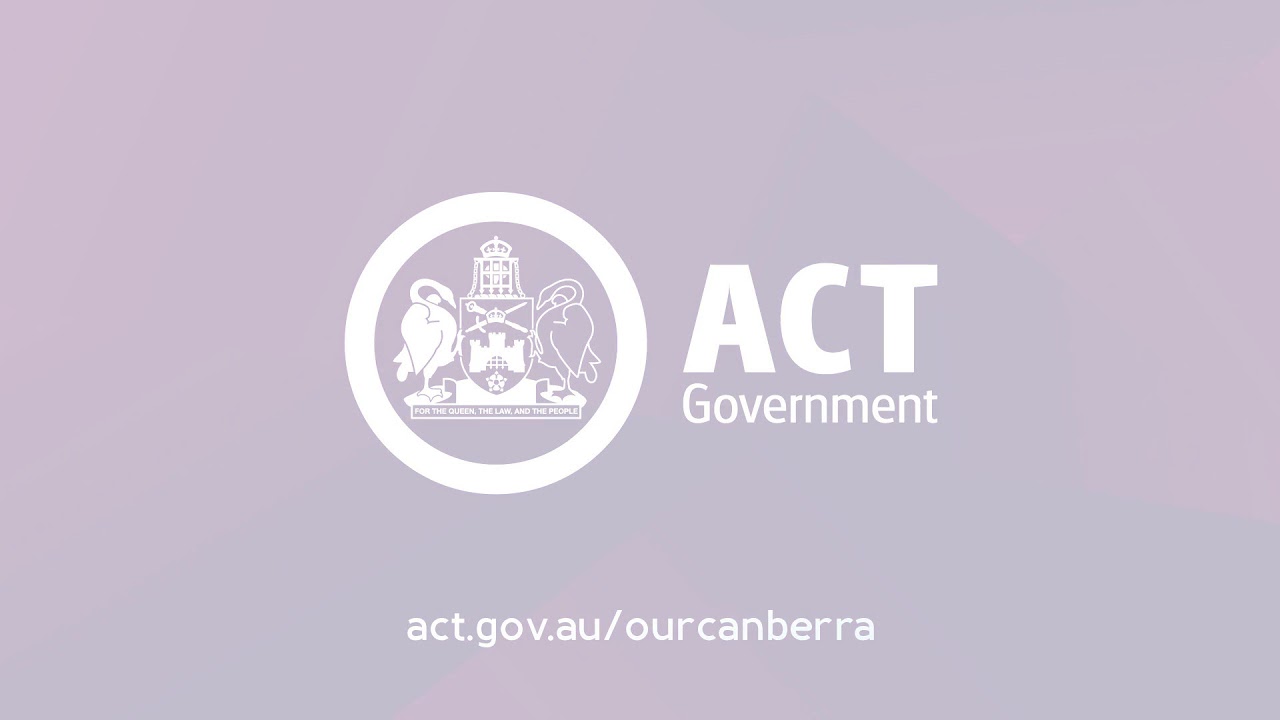The image features a clear, brightly lit sign with a light violet or pale purple background. Central to the image is a white circular seal, which prominently displays two swans—one fully white facing to the right, and one completely purple facing to the left. The swans are outlined in their respective colors. Within this seal, situated between the swans, is a detailed emblem consisting of a castle with a flag, two crossed swords, and a crown or throne at the top. Below the emblem, it reads “For the Queen, the Law, and the People.” To the right of the seal, in large white text, is the phrase "ACT GOVERNMENT." At the bottom of the sign, the website address "act.gov.au/ourcanberra" is displayed, also in white. The overall design is limited to the colors white and purple, emphasizing the contrasting elements in the image.